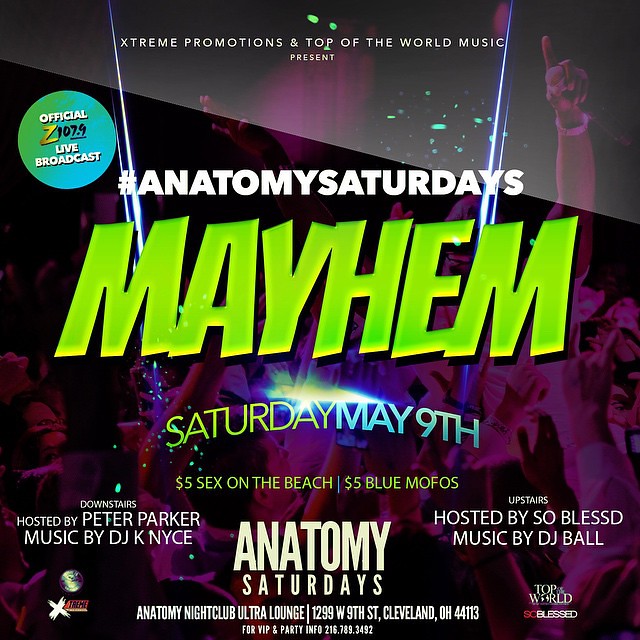This vibrant poster promotes a dynamic entertainment event called "Anatomy Saturdays Mayhem," presented by Extreme Promotions and Top-of-the-World Music. At the top, it proudly advertises an official Z 1079 live broadcast. The event is scheduled for Saturday, May 9th, with a $5 entry fee and $5 drink specials on Sex on the Beach and Blue Mofos. "Anatomy Saturdays" will be hosted upstairs by So Blessed with music by DJ Ball, and downstairs by Peter Parker with music by DJ Nice. The venue for this lively event is the Anatomy Nightclub Ultra Lounge in Cleveland, Ohio, featuring a visually engaging purple background with silhouettes of people dancing, adding to the excitement of the night.